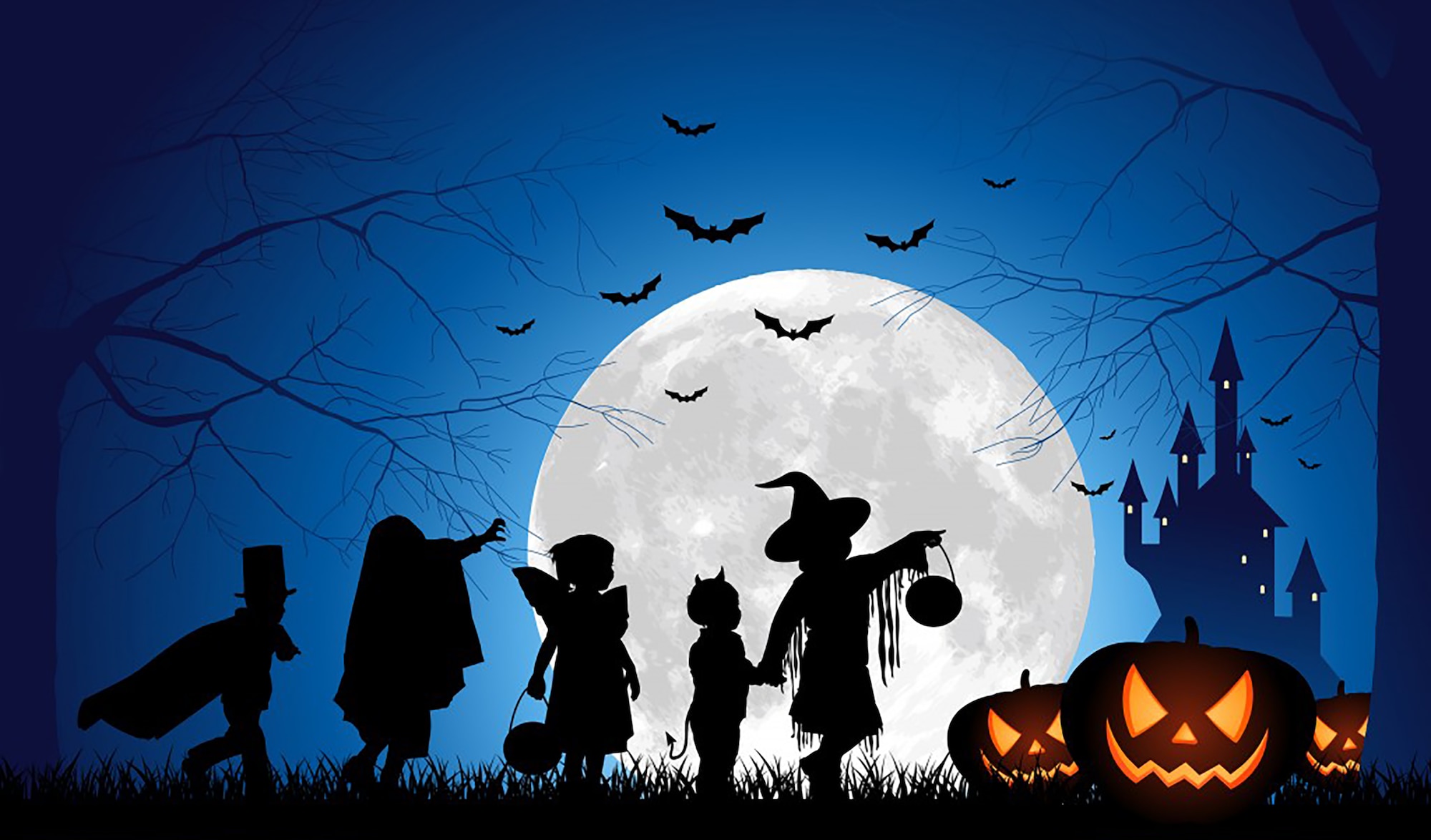In this nighttime vector illustration, the moon, nearly half the height of the graphic, casts a luminous glow in the dark blue sky, highlighting its craters. Silhouetted against this backdrop are five children, each dressed in distinctive Halloween costumes for trick-or-treating. From left to right, you can see a child in a top hat and cloak resembling Dracula, another with a draped sheet like a ghost, one dressed as a magician in a top hat and cape, another as a devil with horns and a tail, and the last with a witch’s hat. They hold pumpkin pails ready for treats. On the ground, three jack-o'-lanterns with glowing menacing eyes and jagged smiles sit amid silhouetted grass. In the distance, a haunted house with glowing windows looms, its eerie presence accentuated by barren trees on either side and bats flying across the sky. The intensifying shades of blue from the moon's illumination to the edges of the image create a stark, haunting contrast perfect for Halloween.